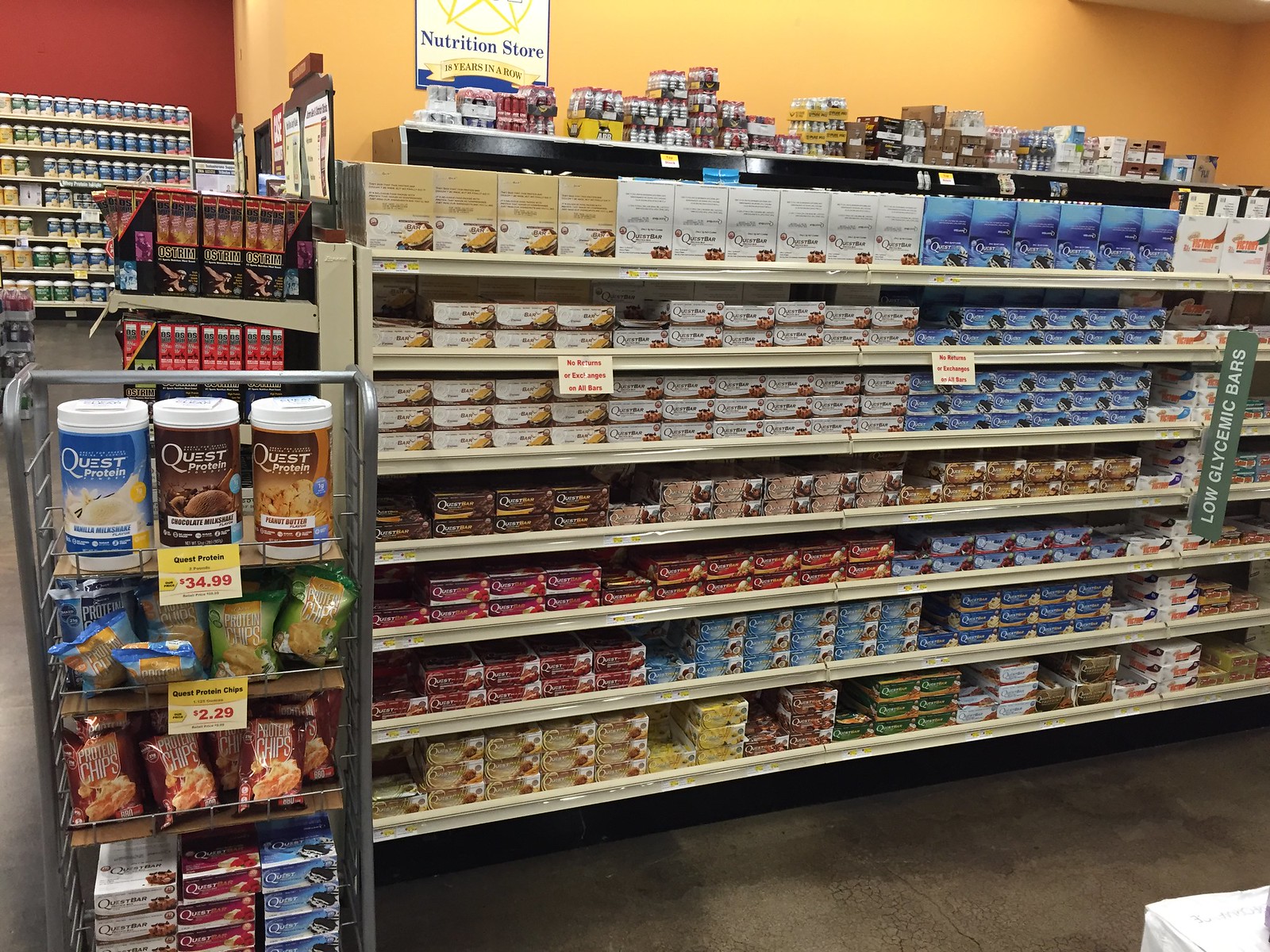The image depicts an indoor scene centered on a door and a set of shelves. The photograph is square in shape and prominently features a tall, tan-colored shelving unit with seven levels. Each level of the shelves is stocked with a variety of items. Behind the shelves, an orange-colored wall serves as the backdrop. Affixed to the wall is a poster that reads "Nutrition Store." The detailed arrangement of the shelves and the inviting color scheme of the wall create a vibrant and organized ambiance within the space.